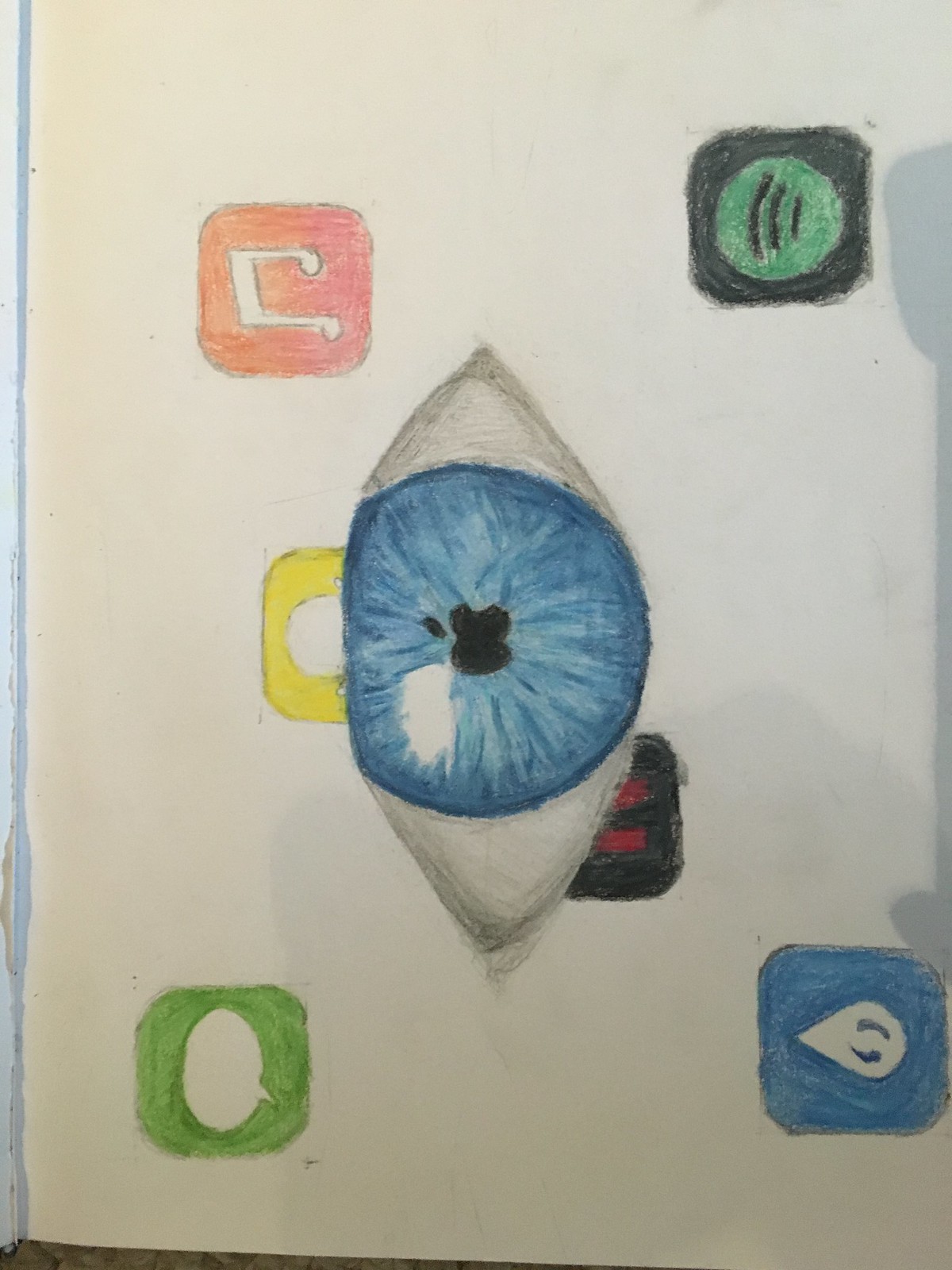This image captures a photograph of a hand-drawn mural on what appears to be a plastered wall. The photograph's authenticity is evident from the glimpse of flooring visible at the very bottom, indicating that the artwork is displayed on a vertical surface. The mural intricately showcases various app icons drawn with meticulous detail. In the top right, there is a hand-sketched representation of the Spotify icon. To the top left, a music app icon is prominently featured. The bottom left corner displays a chat messaging icon, while the bottom right corner features a more abstract design—a white water droplet set against a blue background, with a blue eye and the Apple symbol at its center. The overall impression suggests that this detailed and creative mural may have been a collaborative project, possibly crafted by students.